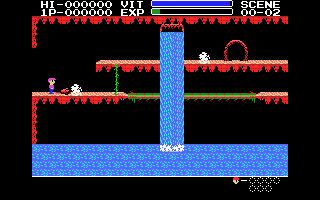In this detailed screenshot from a vintage 8-bit arcade video game, potentially from the 70s or 80s, the upper section of the image features a black background with two lines of white writing filled with zeros. Prominently, it displays "HI," followed by zeros, and "1P" leading more zeros, alongside indicators "VIT" with a blue bar and "EXP" with a barely filled green bar. The text also reads "Scene 00-02" in the upper right corner.

The middle section highlights a pixelated blue waterfall pouring into a body of water below, both rendered in striking blue hues. Two horizontal platforms, displayed against the black backdrop, feature vibrant orange, red, and brown lines. A mystical scene unfolds with a dragon encircled by a ring of fire on the top platform. Below, a figure appears to conversate with the dragon, linked by a green vine that visually connects the tiers. The red lines demarcate these levels, and a distinctive green line climbs between the platforms, adding to the interconnected landscape. This classic shot encapsulates the charm of early video game design, resonating with nostalgic adventure aesthetics.